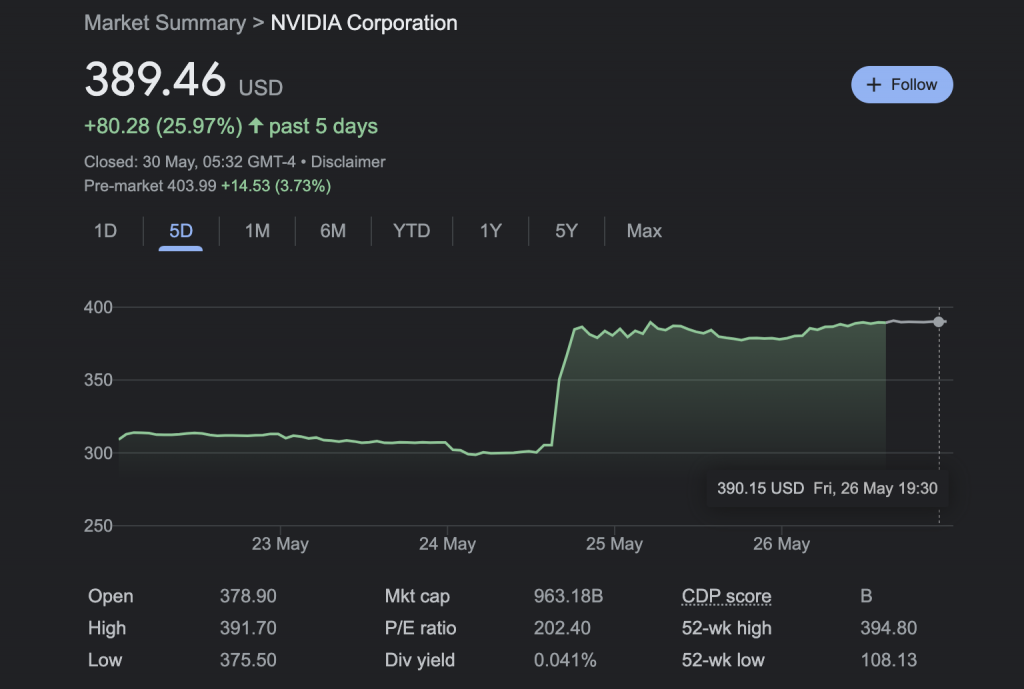Screenshot of a Financial Website Displaying NVIDIA Corporation Stock Market Data

The screenshot appears to be taken from either a website or a tablet, displaying a simple page with a black or dark charcoal gray background and white text. In the upper left corner, there is a heading in pale gray text that reads "Market Summary → NVIDIA Corporation". The company name "NVIDIA Corporation" is written in bright white capital letters.

Below the heading, there is a series of stock market information readings, presented in various color codes for better distinction:
- The primary stock price is shown in white: "389.46 USD".
- Below that, in pale green print, there is a note on its change: "+80.28 (25.97% past five days)".
- Additional information includes: "Closed: 30 May, 5:32 GMT-4" followed by a disclaimer, and data for the premarket: "403.99 +14.53 (3.73%)".

The screenshot also features a graph, depicted in pale green, showing the stock trends. The graph line is shaded lightly underneath, hovering around specific values:
- Numerical values along the Y-axis include: 400, 350, 300, and 250.
- The graph shows a trend starting a bit over 300, dropping close to 300, then sharply rising to around 400. It looks like this trend extends over a five-year timespan, maintaining a high rate towards the end.

At the bottom of the page, there's a column listing various financial metrics such as:
- Open
- High
- Low
- Market Cap
- PE Ratio
- Dividend Yield (Div Yield)
- CDP Score
- 52-Week High
- 52-Week Low

Each metric has specific numerical data beside it corresponding to the overall financial summary and graph. 

Additionally, a blue "Follow" button is located in the upper right corner of the page for users who wish to track NVIDIA Corporation's stock performance.

This detailed display offers a comprehensive snapshot of NVIDIA Corporation's recent stock market performance and history.